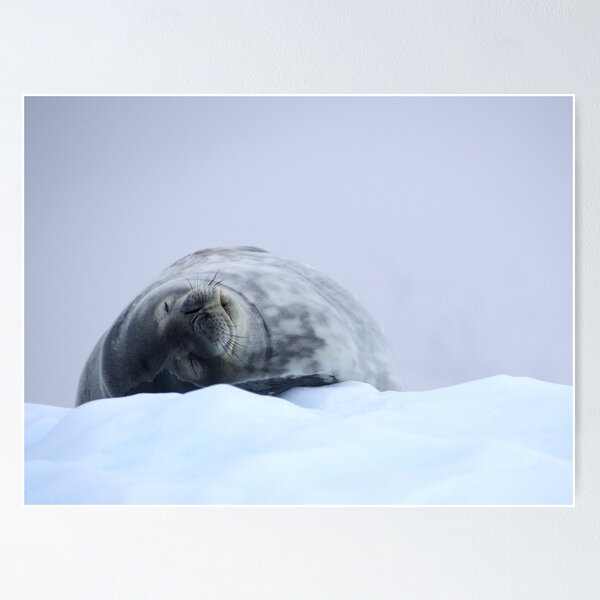In this photograph, we see a very cute, plump baby seal laying on its side on a fresh bed of icy snow. The seal, with its mottled coat of white, black, and gray spots, has its eyes closed as it appears to be sleeping peacefully. The scene is dominated by a light-hued gray, white, and black color palette. The seal's small flipper is tucked under its head, with just the top visible above the snow. Its face is tilted slightly to the right, pointing towards the viewer. The background sky blends seamlessly with the snowy landscape and mirrors the color gradient of the surface upon which the photograph is placed. There is a narrow white frame around the photo, which appears to be against a solid white wall, enhancing the overall serene and minimalist aesthetic of the image.